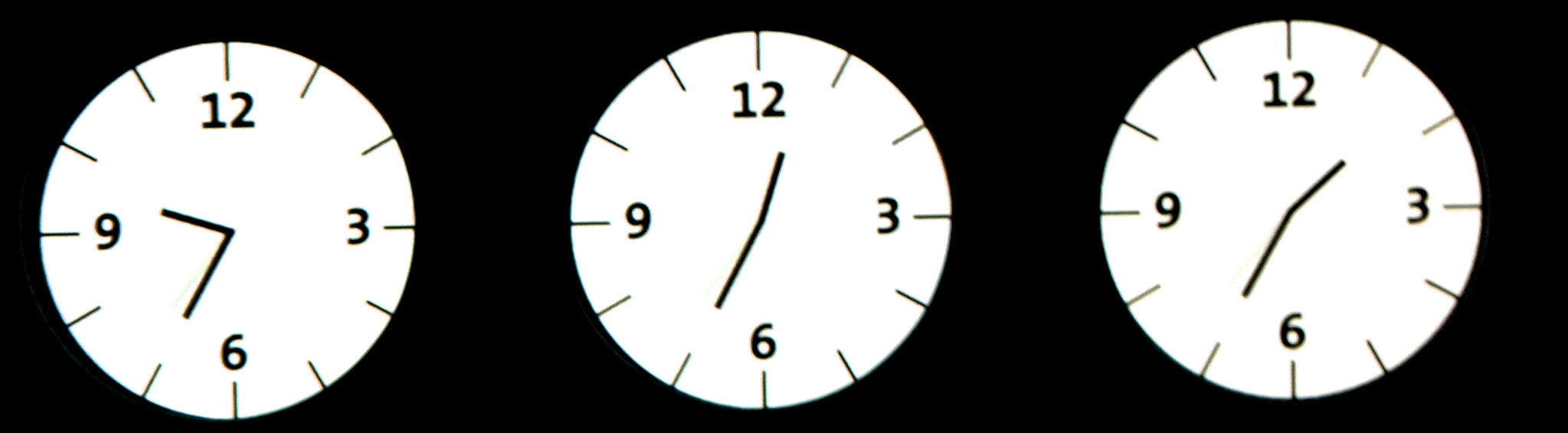This digital illustration features a narrow, horizontal black rectangle as a background, centered on which are three white, round clock faces. Each clock face is detailed with black markings and displays the numbers 12, 3, 6, and 9, with the remaining hours represented by black slashes. The clocks lack second hands, each featuring only hour and minute hands which are also black. The first clock on the left indicates 9:35, the middle clock shows 12:35, and the clock on the right displays 1:35. The overall design is minimalist, with no additional text or elements present.